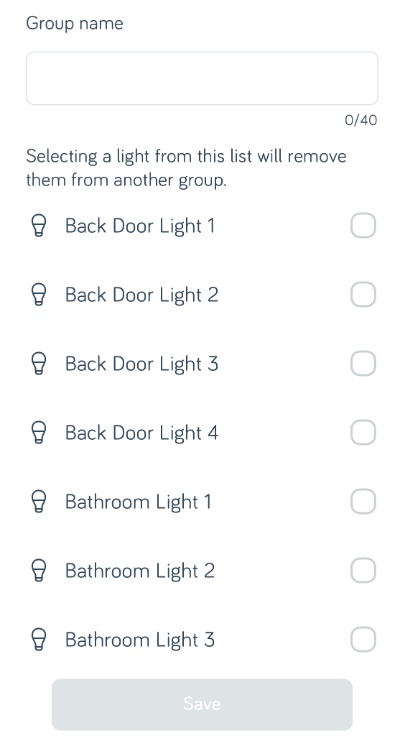This image is a screenshot of a smart lighting control app interface. At the top left, there is the label "Group Name" above an empty rectangular text box where users can input a name for their lighting group. In the bottom right corner of this text box, the characters "0/40" are displayed, presumably indicating a character limit. Centered at the top is a warning message: "Selecting a light from this list will remove them from another group."

Below the message is a list of seven lights, each accompanied by a small light bulb icon to the left and a checkmark box to the right. The lights are identified as follows:
1. Backdoor Light 1
2. Backdoor Light 2
3. Backdoor Light 3
4. Backdoor Light 4
5. Bathroom Light 1
6. Bathroom Light 2
7. Bathroom Light 4

At the very bottom center of the image, there is a "Save" button in white text on a gray background.